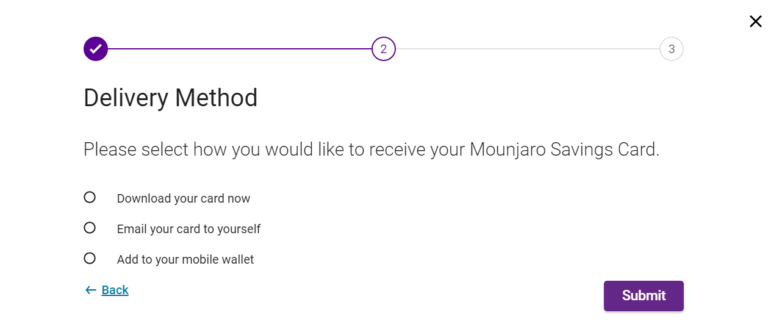The web page features a predominantly white background with various key elements. At the top, there is a dark purple circle containing a white check mark. A purple line extends from this circle to another circular element, which is white with a purple border and a purple dot in the center, appearing like a three-dimensional tube. Adjacent to these circles, there is a gray section featuring a gray numeral "3" within a circular border.

Below these graphical elements, a header in bold black text reads, “Delivery Method.” Underneath, a subtext in gray provides instructions: “Please select how you would like to receive your Mounjaro savings card.”  

Three bullet points follow, each marked by a white circle with a black border:
1. "Download your card now."
2. "Email your card to yourself."
3. "Add your mobile wallet."

On the left-hand side beneath this list, there is a cyan-blue arrow pointing left, accompanied by the word “Back” with a capitalized and underlined "B". 

In the top-right corner of the web page, a black “X” is positioned for closing the interface. At the bottom right, there is a dark purple button labeled "Submit" in white text. 

No additional details are present on the web page.